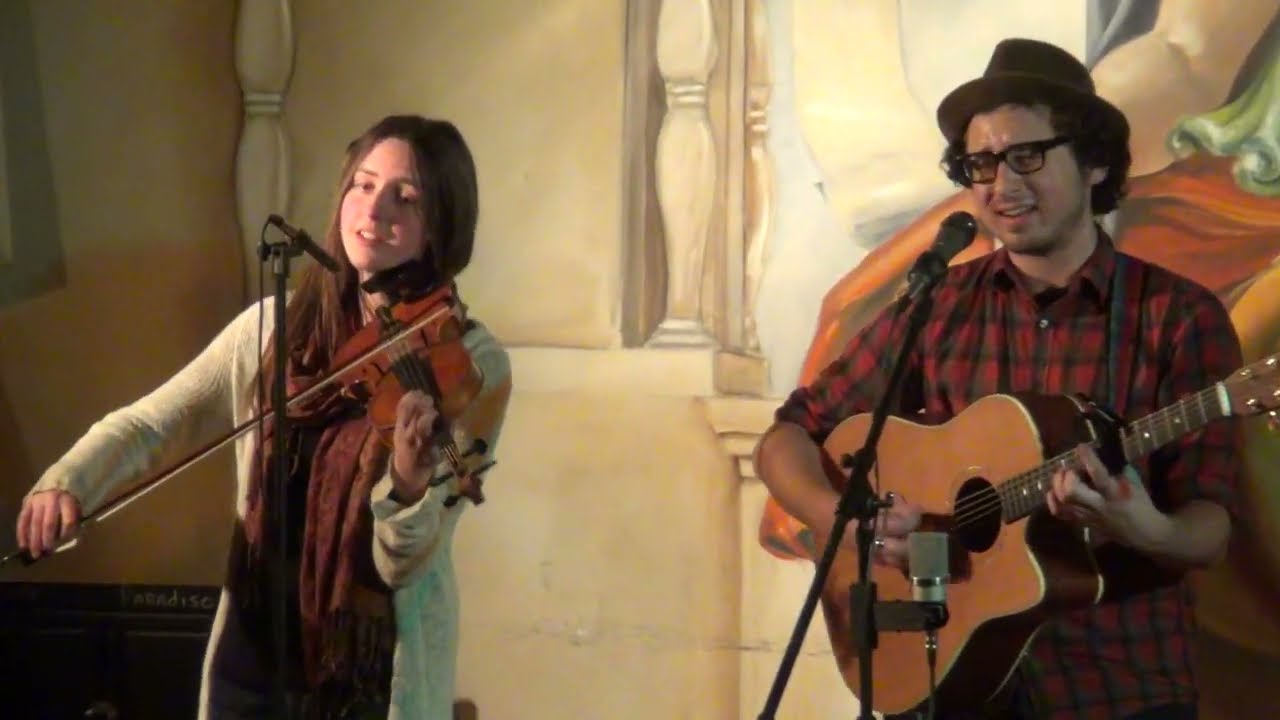In the image, three musicians are performing live on stage, framed by an audience and a background mural. On the left, a female violinist wears a white sweater over a maroon shirt, blue jeans, and brown boots. She has long brunette hair and stands next to a piano with items on its bench. A microphone is set up in front of her. In the middle, a man plays a light brown acoustic guitar with a strap. He sports a red and black flannel shirt, blue jeans, brown shoes, and a brown hat, complemented by black nerd glasses. His microphone is also visible. To the right, a man in a black sweatshirt, black pants, and a yellow beanie plays an upright bass made of tan-colored wood. He faces the other musicians while they face the audience. The audience is seated and in shadow. The background features a mural depicting a person in an orange robe and a green shirt, reminiscent of an ancient or religious figure. Scattered musical equipment is visible on the left side of the stage, enhancing the detailed setting of this dynamic live performance.